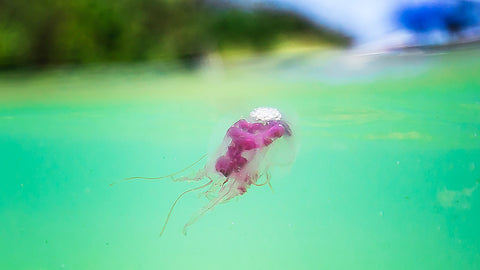This captivating image, taken by a photographer, features a striking pink and purple jellyfish, partially submerged underwater. The photograph, a focused close-up, highlights the jellyfish’s translucent, globe-shaped body with intricate, rope-like internal structures, and its delicate, waving tentacles. The jellyfish’s outer casing is see-through, revealing a mesmerizing fuchsia pink hue that stands out prominently. The water around the jellyfish, a blend of greenish blue and light turquoise, creates a tranquil ambiance. Despite the blurry background, one can make out the faint outlines of trees, a beach with sand, and portions of the sky with clouds, suggesting a tropical setting where part of the camera was submerged to achieve this unique perspective. The hyper-focused lens emphasizes the ethereal beauty of the jellyfish amidst its serene aquatic environment.